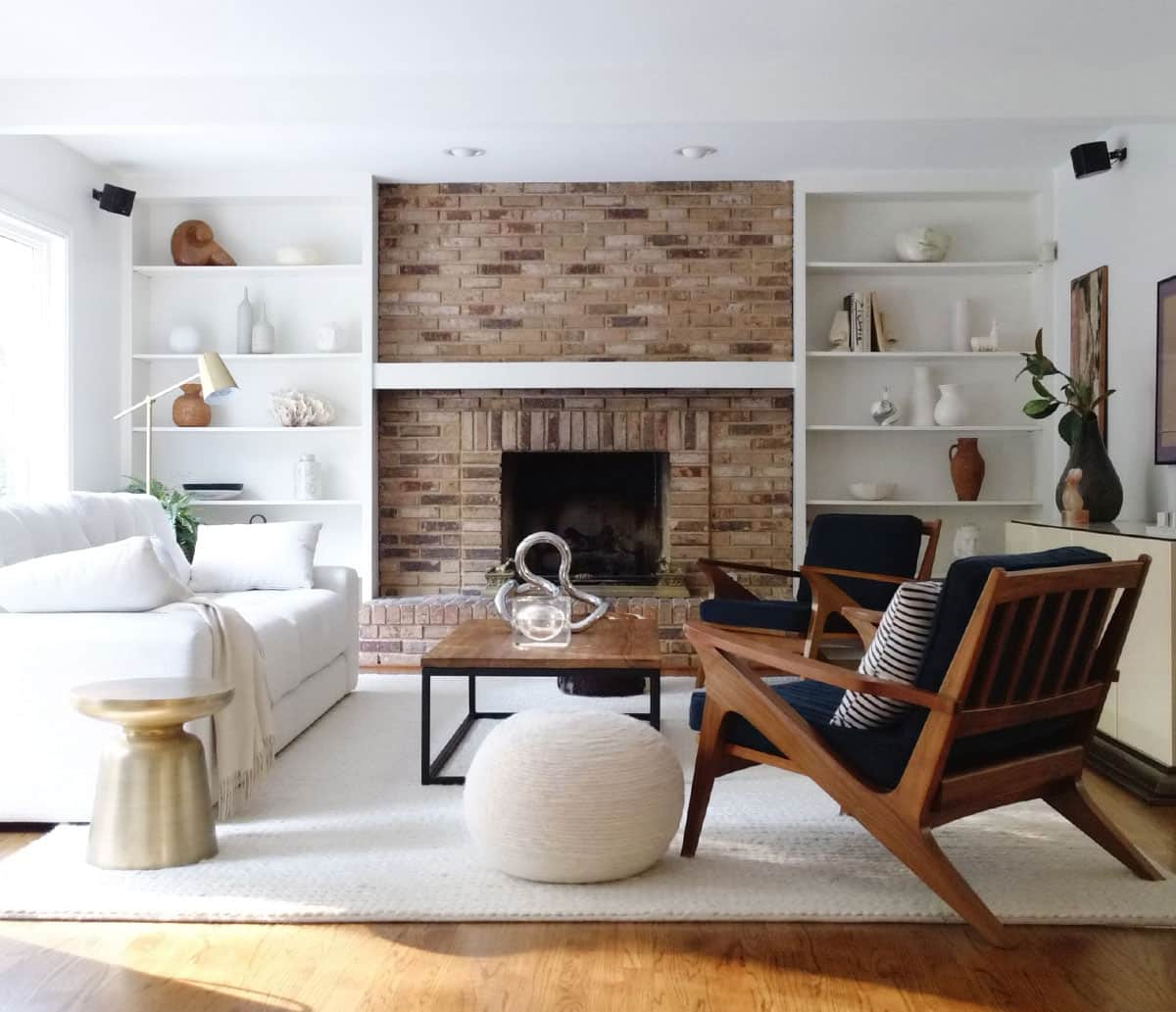The living room depicted in the photograph exudes a harmonious blend of modern and rustic styles, creating a cozy yet elegant atmosphere. The walls and ceiling are a pristine white, enhancing the room's brightness, which is further amplified by a large unseen window on the left that fills the space with natural light. The focal point of the room is a substantial brick fireplace framed with light, bronzed bricks, topped by a white mantle. Flanking the fireplace are built-in white bookcases adorned with a variety of white and wooden decorative elements, including vases, white coral, pottery, and a piece of art.

On the left side of the room, a large, plush white sofa sits cozily in front of the window, accompanied by a gold-colored brass side table. Complementing the sofa, two dark wooden lounge chairs with navy blue cushions are positioned on the right, one of which features a stylish navy and white striped pillow. Between these seating arrangements, a modern coffee table with a brown wooden top and black metal legs provides a central gathering spot, displaying an artistic sculpture resembling a stylized bird or snake.

The hardwood floor is partially covered by a creamy white area rug, contributing to the room's warmth and cohesion. Adding to the seating options, a fuzzy white ottoman, resembling a miniature bean bag, sits beside one of the lounge chairs. The decor is punctuated by subtle lighting elements positioned around the room, ensuring a cozy ambiance during the evenings. Overall, this inviting living room masterfully balances clean, modern design with rustic touches for a timeless and comfortable feel.